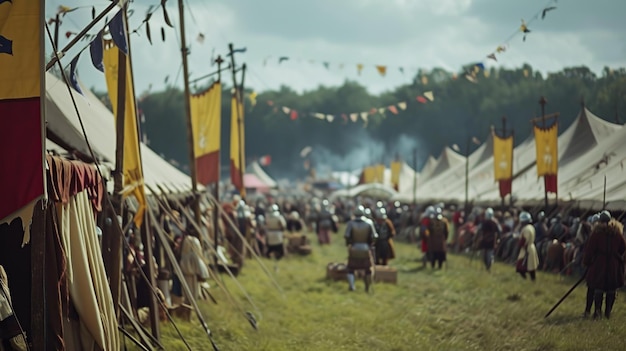The photo captures a vibrant outdoor renaissance fair, bustling with life under a sunny sky. Beige hand-canvassed tents line both the left and right sides of a grassy clearing, each adorned with medieval-style flags. These flags are visible atop posts, three on each side, boasting a distinct yellow top and an orange-cranberry bottom with an indecipherable logo. Above the scene, multicolored triangular streamers flutter in the breeze, adding to the festive atmosphere. In the mid-ground, people dressed in steel armor, complete with metal helmets, gather and engage, possibly reenacting medieval scenarios. A horse can be spotted in the lower right-hand corner, though it is unclear if it is being ridden or led. The furthest backdrop reveals a tree line and hints of smoke, possibly from a cookout, suggesting the presence of food vendors likely scattered among the tents, enhancing the medieval ambiance of the fair.